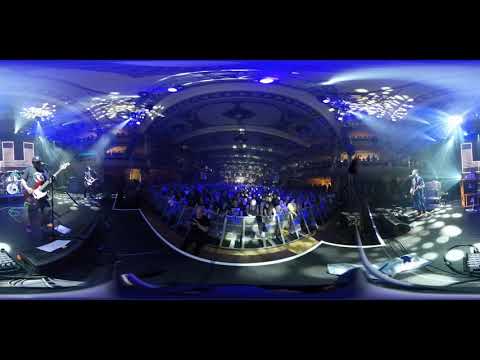This photorealistic image, albeit of poor resolution and with details difficult to discern, appears to have been captured with a 360-degree camera, resulting in significant warping. Depicted is a large, indoor concert hall characterized by its dark ambiance and extensive lighting effects. Dominating the scene is a well-lit stage with a black floor, flanked by two performers. 

On the right side, a musician sits in front of a microphone with what seems to be a guitar or string instrument, illuminated by numerous blue and bright ceiling lights, and accompanied by dotted floor lights that enhance the stage's vibrant atmosphere. On the left, another performer stands in front of a black microphone, holding a guitar, and dressed in a gray shirt and hat. 

Central to the image is the audience, situated behind a white fence, rendered in hues of blue owing to the stage lights. The crowd is largely indistinct due to the image’s low resolution, but it’s clear that they fill a considerable and deep space within this concert hall. The panoramic nature of the shot introduces distortion but also captures the extensive room with its possible curved ceiling. Additional elements like speakers and possibly other instruments are visible, contributing to an immersive concert-like setting. The entire scene features a dynamic interplay of light beams on the ceiling and floor, enhancing the overall concert atmosphere.